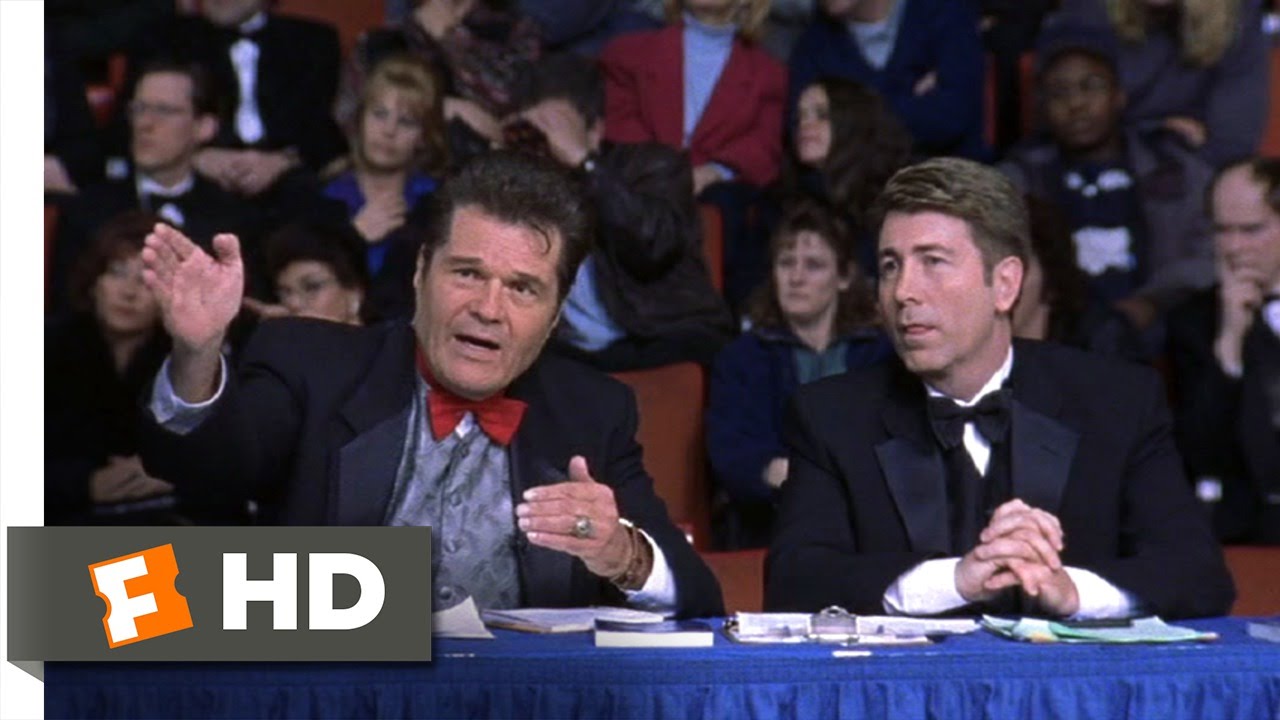The image shows two men, likely commentators or judges, seated at a narrow table draped with a blue tablecloth. Both have clipboards and notes spread before them. In the background, there is a sizable audience seated in stadium-like, orangish chairs. The crowd includes a mix of men and women, with a variety of hair colors and clothing in shades of red, white, and blue. A logo featuring an orange puzzle piece with a white F, followed by "HD," is visible in the bottom left corner.

The man on the left appears to be in his fifties, with short black hair, wearing a navy suit, gray vest, and red bow tie. His left hand, adorned with a ring and a wrist brace, rests on the table, while his right hand is raised as if pointing or explaining something. He looks to be speaking, with his mouth slightly open.

The man beside him, seemingly in his thirties or forties, has short blondish-brown hair and is dressed in a black tuxedo with a black bow tie and white shirt. His hands are folded on the table, and he appears to be attentively listening, looking in the same direction as his colleague.